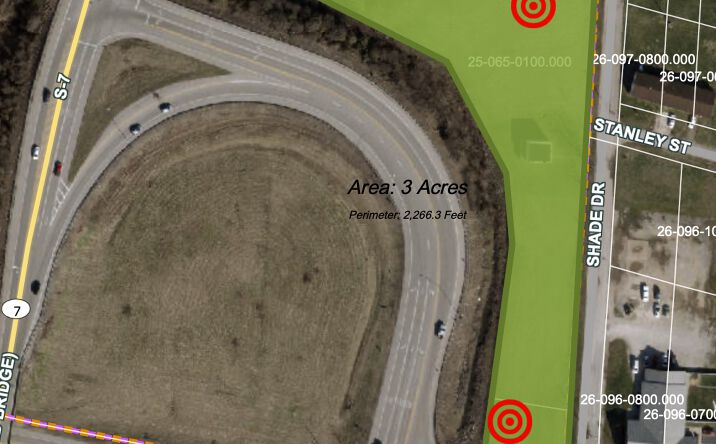The image is a detailed bird's-eye view of a map featuring a mix of natural and urban elements. On the left, there is a circular track or road with a portion cut off at the bottom, accompanied by black text indicating "Area: 3 acres" and "Perimeter: 2,266.3 feet." This area appears to have green grass with several red bullseye-like circles. Adjacent to this, towards the right, is a partial view of a city street map, displaying named streets like Shade Drive running vertically and Stanley Street horizontally. The streets are marked with solid and dashed white and yellow lines, and you can see a mix of vehicles including black, white, red, and gray ones. The background includes some green spaces and buildings. Notable elements include numerical codes like 26-096-0800-000, and an orange and purple striped line. The overall color scheme is a mix of grayscale with highlighted elements in green, yellow, red, and shades of gray.